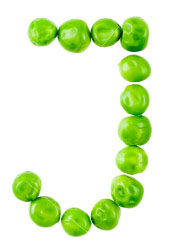The image depicts 13 small, uniformly sized, shiny green peas arranged to form the letter 'J' on a bright white, shadowless background. The peas are divided as follows: four peas line the top horizontally, while the remaining nine curve downward to complete the 'J' shape. Each pea is a vibrant green and appears similarly shaped, giving the impression they might be canned due to their perfect appearance. The letter 'J' formed by the peas stands out clearly against the stark white backdrop, creating a simple yet striking visual.